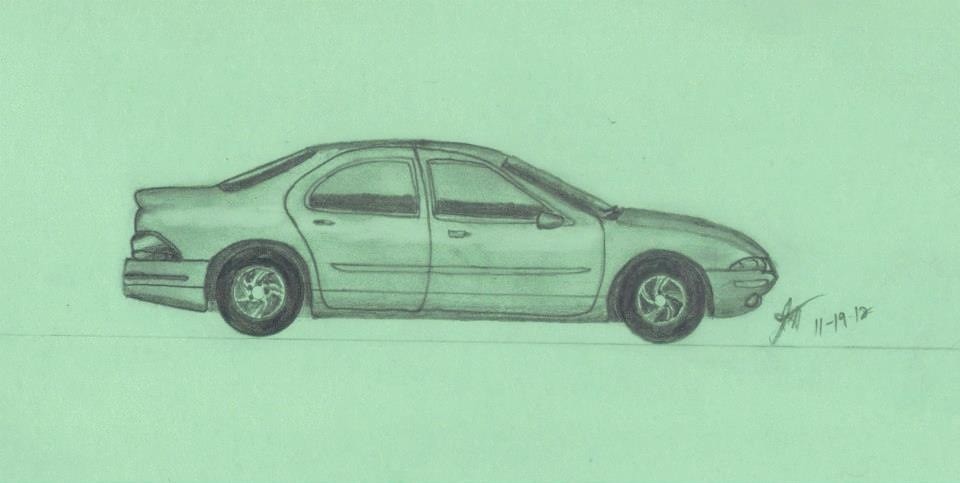This is a highly realistic pencil or charcoal drawing of a four-door sedan on a muted light mint green, long rectangular paper. The car, viewed from its right side, faces to the right and is depicted in meticulous detail without any cartoonish elements. The sedan has small tires with equally-sized hubcaps, a curved rounded nose with a diminutive front bumper, and a small rear trunk with a slightly protruding bumper. A pinstripe runs down the side between the front and back door. The artist's signature and the date "11-19-12" are located near the bottom right bumper of the car. Despite the realism, there are no visible badges or markings that reveal the make and model of the car.